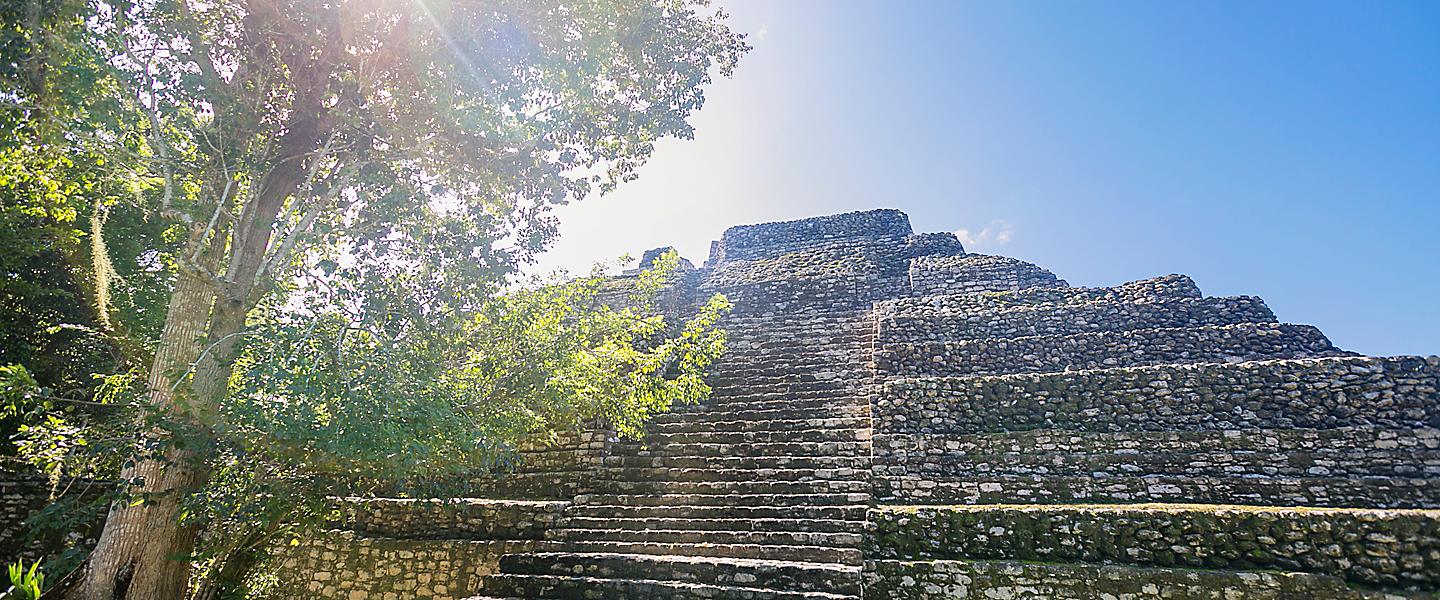The image depicts an ancient archaeological site likely from the civilizations of the Maya, Aztec, or Inca. Located centrally is a grand stone pyramid with steep, wide steps climbing toward the top. These stairs appear heavily weathered and green with moss. A notable feature is the structure at the apex of the pyramid, rising above the rest of the temple. Dominating the left side of the image is a tall tree whose branches and green foliage obscure part of the pyramid, with its trunk extending upwards and branching into two large limbs halfway up. Sunlight filters through this tree, casting a golden hue on some of its leaves and partially illuminating the pyramid. The image is set against a backdrop of a clear, blue sky with minimal clouds, suggesting a bright daytime scene. Overall, the pyramid, with its moss-covered steps and the vivid greenery of the tree, commands the center of the composition, exuding an air of historical mystique and natural beauty.